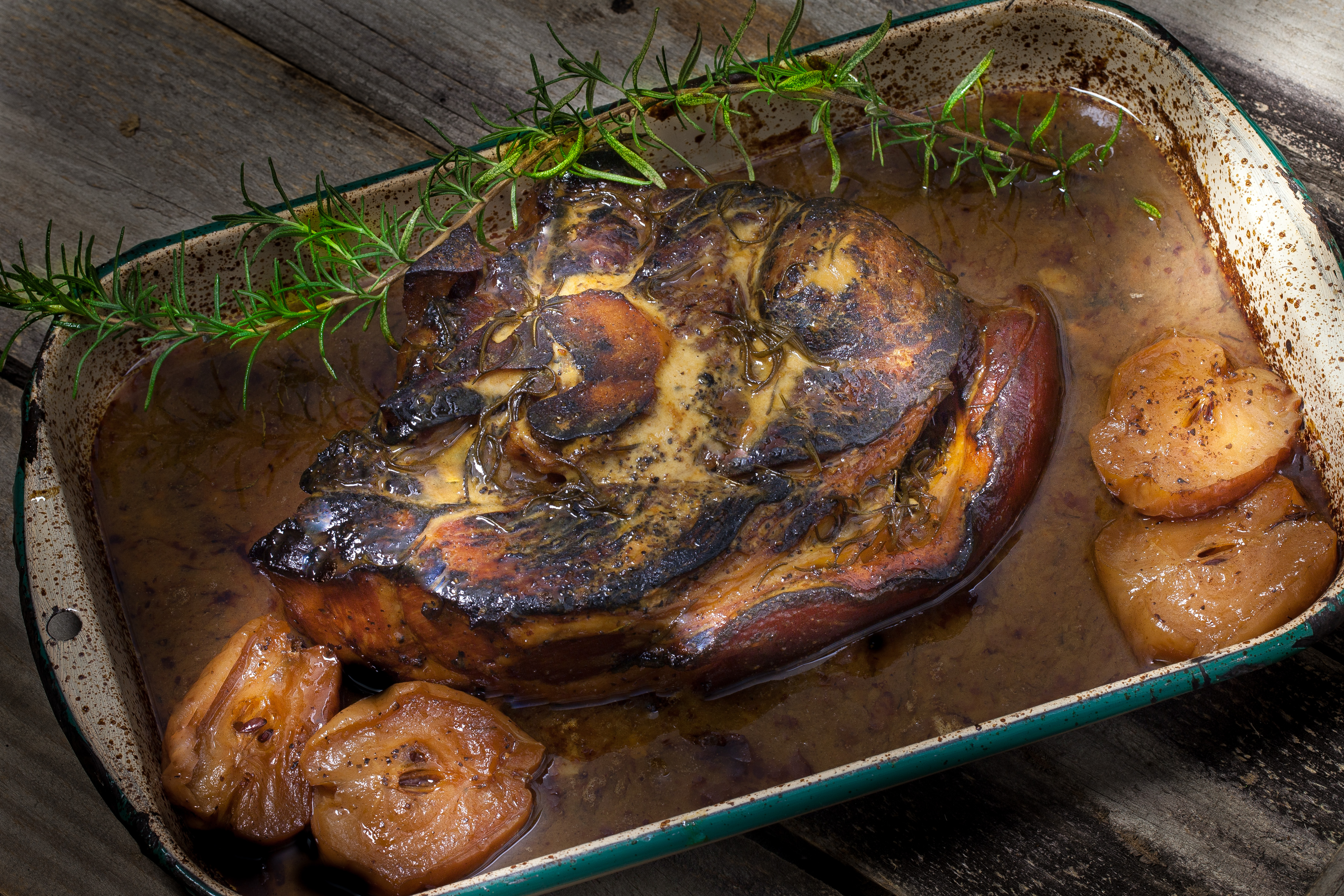The image depicts a close-up view of a rectangular baking pan, likely metal, filled with a savory dish. The pan, speckled and splattered with burnt residue, rests on a dark, grayish wooden surface, possibly a picnic table outdoors. At the center of the pan lies a huge, thick steak with a charred top, exuding yellow-colored fat buildup, indicating it has been sitting after cooking for a while. The steak is surrounded by a watery, brown gravy or juice. Four browned apple slices, or possibly potatoes, are neatly positioned with two on the left and two on the right of the pan. Resting above the steak is a long, slightly cooked, green sprig of rosemary. The overall presentation suggests a hearty, rustic meal, perhaps prepared for an outdoor gathering.